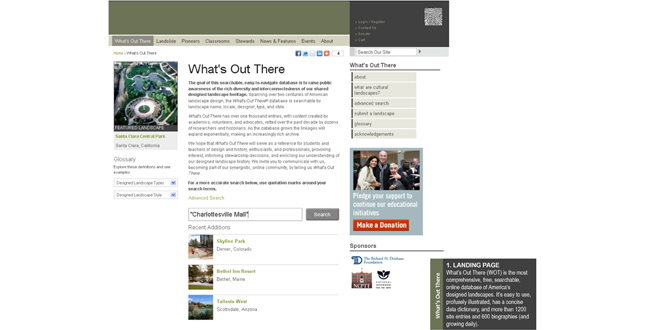A blurry screenshot of a website showcases a layout that becomes increasingly indistinguishable upon zooming in. At the top of the page, a light brown horizontal bar spans from the left to the right. Adjacent to it on the right side, a dark brown rectangular section contains some small, illegible white text and what appears to be a QR code. Below this header, a series of menu items stretch across the page, though their details are obscured due to the blurriness. Further down the page, a white section features an aerial photograph of a building surrounded by trees. To the right of this image, there is additional content that remains unreadable in the screenshot.